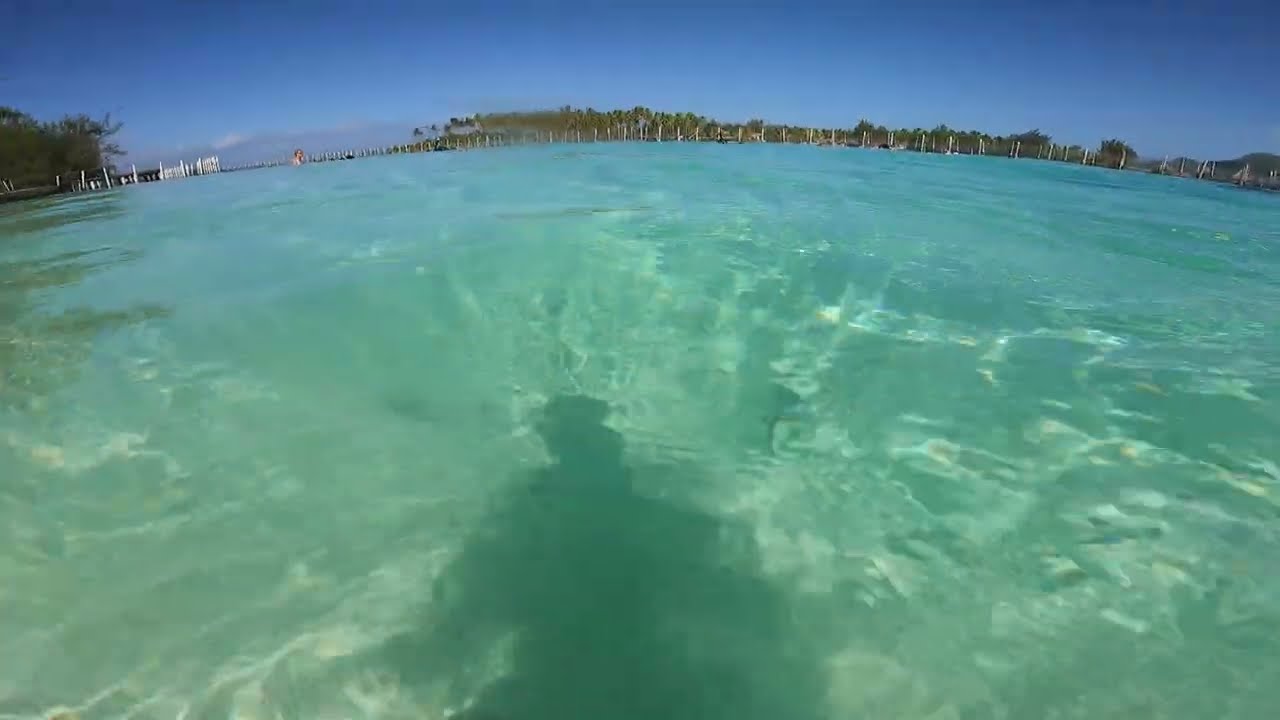In this captivating panoramic photograph, the primary focus is on the stunning turquoise-green water that occupies the majority of the frame. The image appears to be taken from a first-person perspective, as evidenced by the shadow of the photographer at the bottom center. The serene water is a blend of green and blue hues, with subtle reflections that create an almost mesmerizing effect. Toward the far left, a person stands shoulder-deep in the water, adding a touch of human presence to the tranquil scene.

On the far right, sailboats can be seen dotting the water, contributing to the picturesque coastal ambiance. In the distance, a blurred, possibly shadowed land encompasses feathery green foliage and a low hill off to the left. The distant shoreline features a possible fence line or docks, though specific details are indistinguishable. Notably, near the left side of the image, a white dock or bridge extends into the water, accompanied by white pylons.

The upper portion of the photograph frames a beautifully clear blue sky, with very few clouds visible off to the left. The overall scene captures a peaceful moment, highlighting the natural beauty of the water, shoreline, and sky.